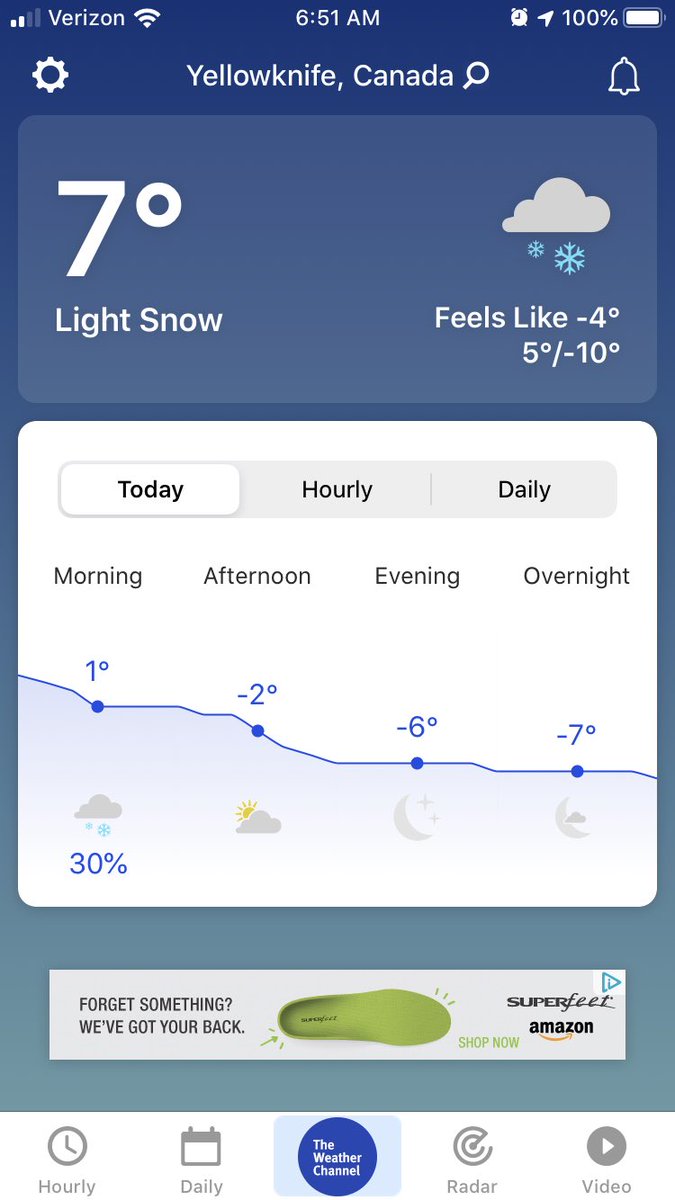The screenshot depicts a weather app interface with a gradient background transitioning from blue at the top to greenish-blue at the bottom. The text is rendered in white. 

At the top of the screenshot, the status indicators show the signal strength, a white spot signal indicating connectivity, the current time displayed as 6:51 AM, a clock icon, and a fully charged battery at 100%. An upward diagonal arrow icon is present, along with a settings icon. The location is identified as Yellowknife, Canada, with accompanying search and notification (bell) icons.

Below this header, a rectangular section with a cornflower blue background contains the current weather details: "7 degrees, light snow," alongside a graphic of a cloud with snowflakes. It also mentions that it "feels like -4 degrees" despite the actual temperature range being "5 degrees to -10 degrees."

Further down, a white box features three tabs labeled "Today," "Hourly," and "Daily." The "Daily" tab breaks the forecast down into segments: "Monday, Afternoon, Evening, Morning, Afternoon, Evening, and Overnight," with a line chart indicating temperature changes. The chart starts at 1 degree in the morning and drops to -7 degrees overnight.